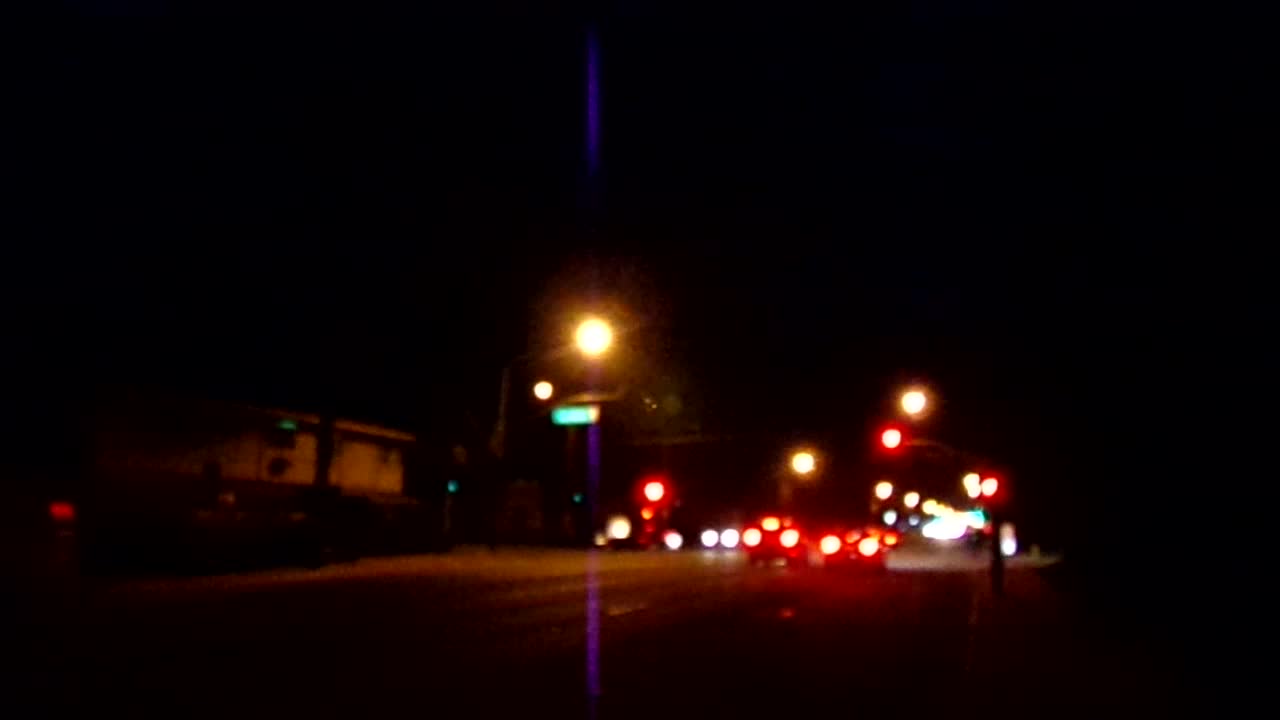This nighttime landscape photograph, captured in landscape orientation, showcases a scene filled with intriguing elements and subtle details. The background is heavily blurred, creating a dreamy ambiance where numerous street lights shine ethereally through the haze. On the center left of the frame, a two-story white building stands with an awning adorning its front, offering a quaint architectural detail.

Dominating the composition are two captivating purple flashes of light, descending vertically in the center of the image. Nestled between these luminous purple streaks is a prominent area of bright white light, casting beams that extend outward from its core. This intense illumination creates a focal point that draws the eye.

Additionally, street lights hang above the road, their soft glow contributing to the overall serene mood. To the center-right of the photograph, the taillights of several cars can be seen, their red hues creating a dynamic contrast as they trail up the road, adding a sense of movement to this tranquil nighttime scene.